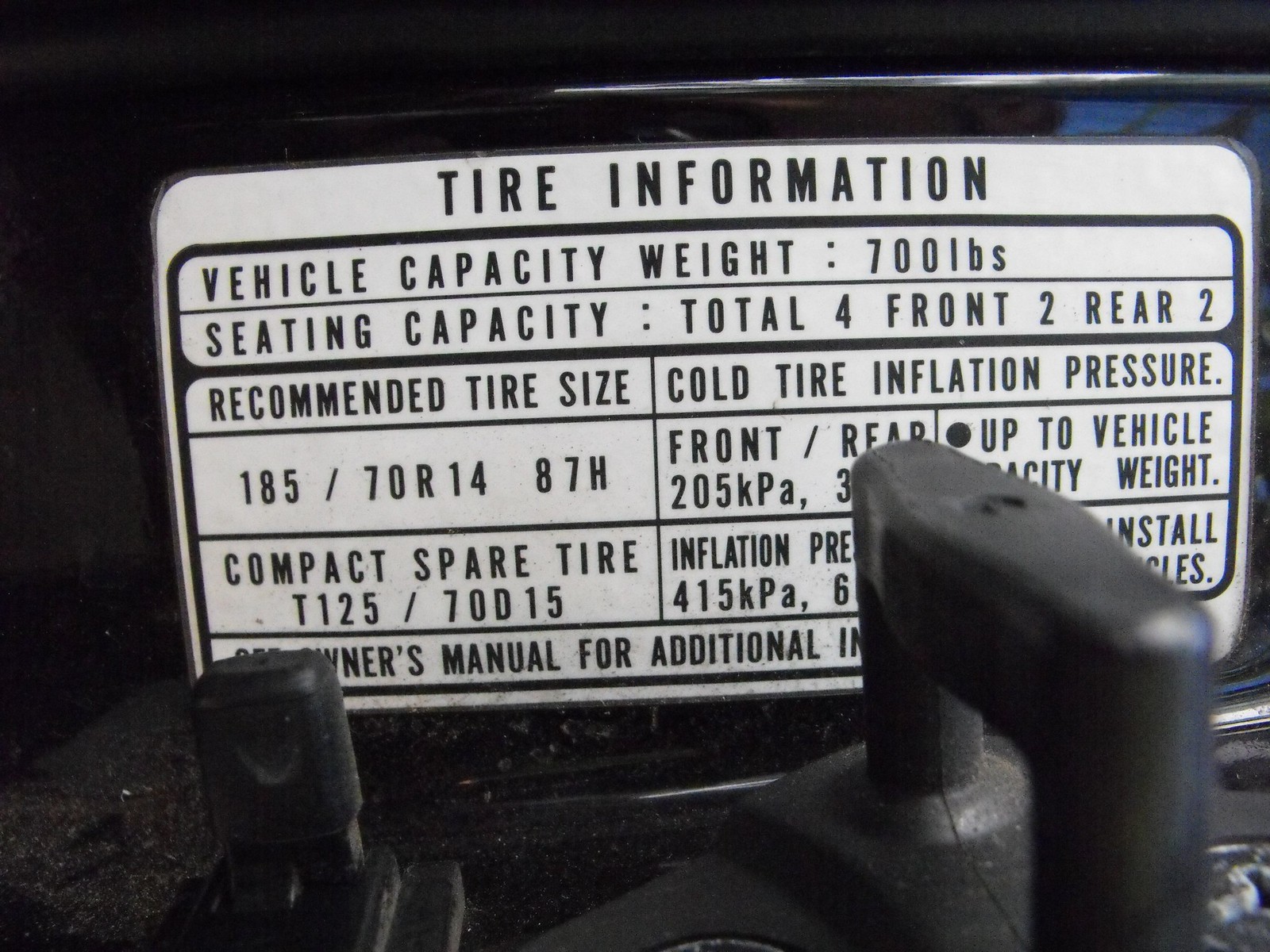This image captures a close-up view of a white, rectangular tire information placard with rounded corners and a black border, located inside a vehicle. The sign prominently displays essential details about the vehicle's tire specifications and capacity. The top of the placard reads "Tire Information," followed by "Vehicle Capacity Weight: 700 lbs" and "Seating Capacity (Total: 4, Front: 2, Rear: 2)." Below, it specifies the "Recommended Tire Size: 185-70R14 87H" and "Cold Tire Inflation Pressure (Front: 205 kPa, Rear: hidden by a black knob)." It also mentions "Up to Vehicle Capacity Weight" and "Compact Spare Tire: T125-70D15, Inflation: 41 kPa," although part of this information is obscured by a foreground black knob. The placard looks somewhat like a license plate and is surrounded by parts of the engine, including tubes and black handles. The background mostly fades into darkness with a little hint of blue, making it challenging to discern further details.